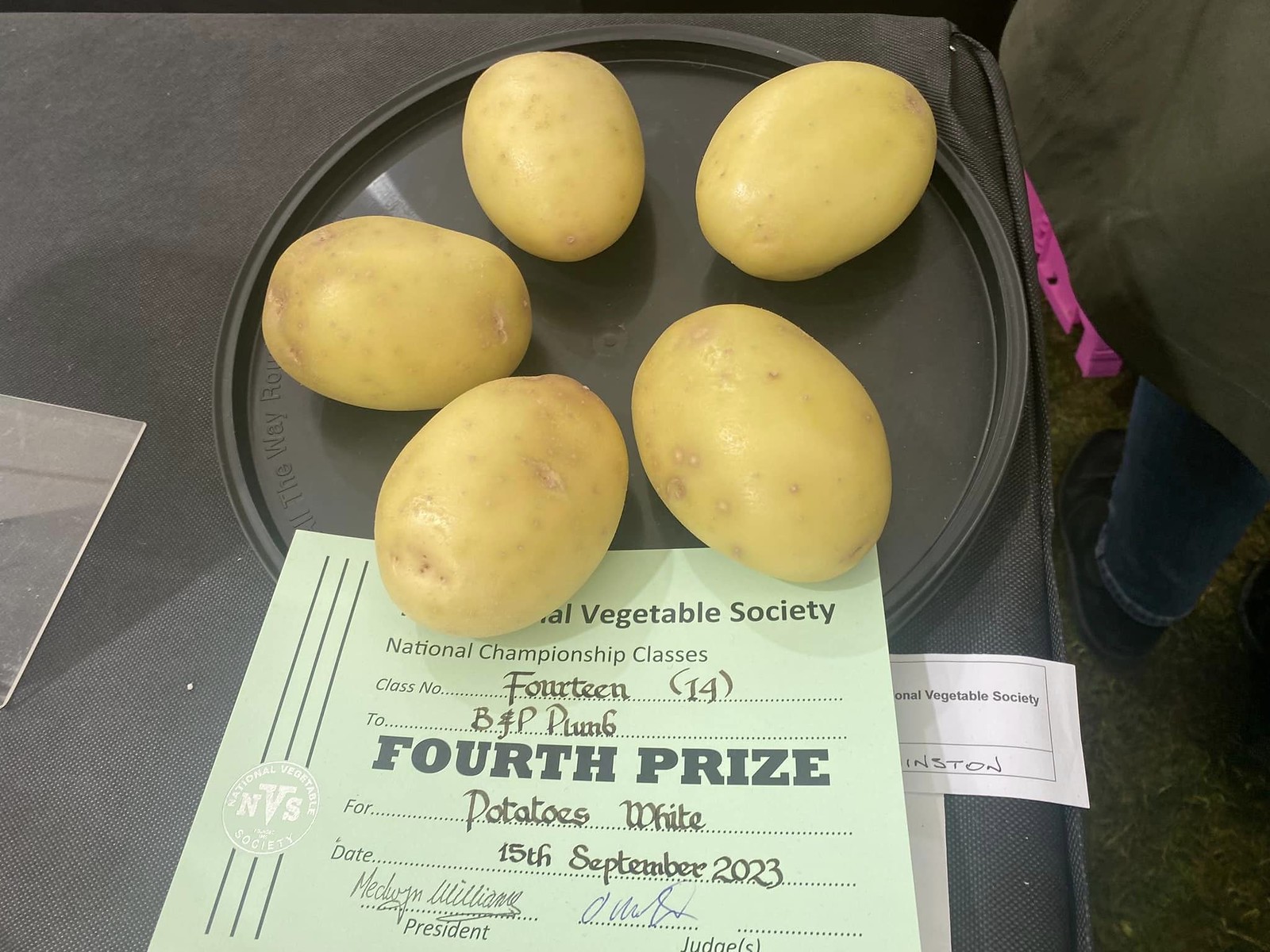The image depicts a black circular plate with five yellow (or white) potatoes meticulously arranged in a star shape: one at the top, one on the right, one on the left, one on the bottom left, and one on the bottom right. This plate is part of a vegetable contest, as indicated by the green paper beneath it, which reads "Vegetable Society National Championship Classes." Specifically, it mentions "Class Number 14" and "Fourth Prize for Potatoes White," dated 15th September 2023. The green paper also bears signatures from the judge and the president of the Vegetable Society. In the background, part of a table is visible, indicating the setting of the contest.